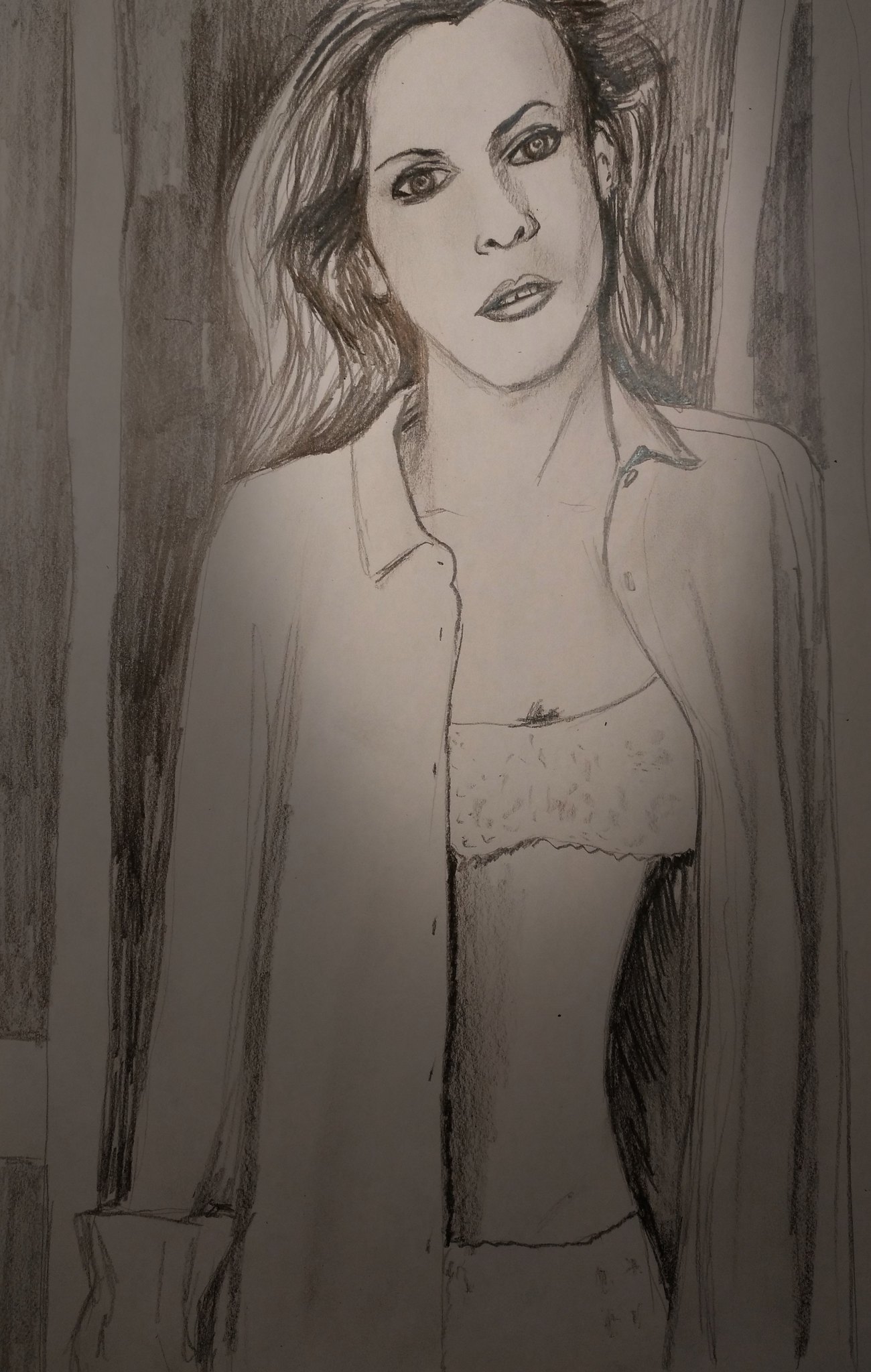In this detailed pencil sketch on a cream-colored background, a striking female figure is captured. She wears a small tube top or bra beneath a long-sleeved, collared shirt, left open to reveal her midriff. Just above the tube top, there’s a dark marking indicative of a tattoo, though its design is not discernible. Her face, framed by long, thick, wavy hair cascading past her shoulders, features large, light-colored eyes and thin eyebrows. Her expression is poised and enigmatic, drawing the viewer’s attention. The background is a vertically striped wall, adding a structured contrast to the fluidity of her hair and attire. The meticulous pencil strokes provide texture and depth to the composition, giving it a raw and evocative quality.